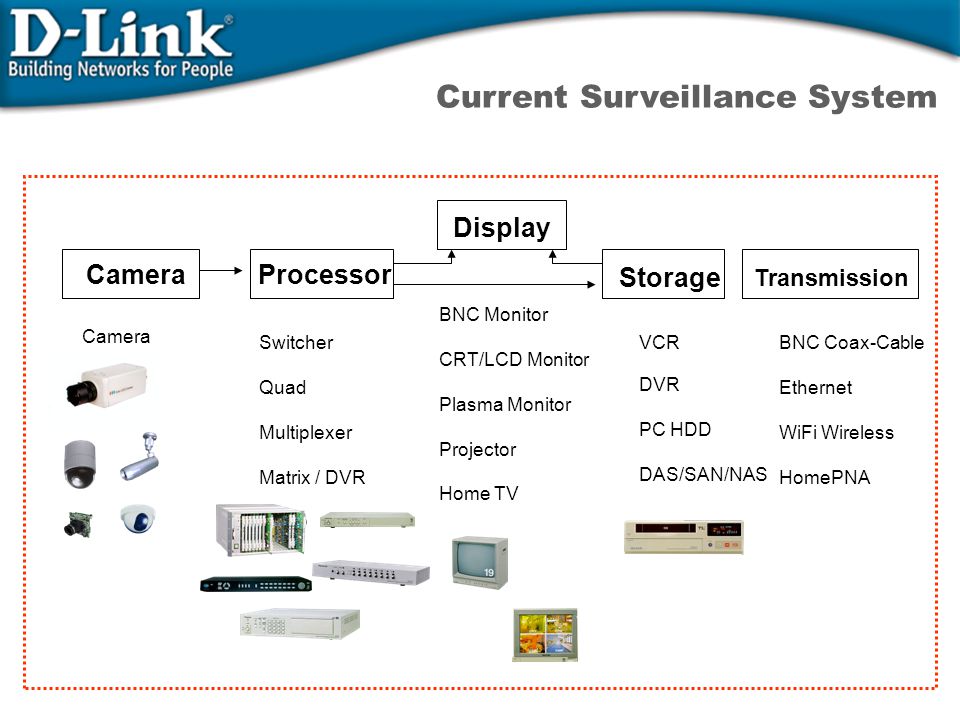The image displays a slide from a PowerPoint presentation on a white background, adorned with text and small images detailing a surveillance system overview. At the top left-hand corner, it reads "D-Link" in large white letters, followed by the tagline "Building Networks for People." On the right side of this header, in dark gray text, it states "Current Surveillance System."

Below the header, the main content is encased within an orange dotted border. Inside this border, the top left features the word "Camera" in a rectangular box, with an arrow pointing right to another rectangular box labeled "Processor." The "Processor" box has two arrows: one pointing right and slightly upwards to a box labeled "Display," and another pointing left to a box labeled "Storage." Additionally, an arrow connects "Storage" to "Display," and on the right side of "Storage," there is a "Transmission" box.

Each rectangular box contains specific items related to its category, illustrated with text and images. Under "Camera," there are various camera types depicted: webcams, larger cameras, and security cameras. "Processor" includes terms like Switcher, Quad, Multiplexer, Matrix, DVR, accompanied by their images. The "Display" box lists and shows items such as BNC Monitor, CRT, LCD Monitor, Plasma Monitor, Projector, and Home TV. For "Storage," there are VCR, DVR, PC, HDD, and DAS/SAN/NAS devices, each illustrated. Finally, "Transmission" details BNC, Coax Cable, Ethernet, Wi-Fi, Wireless, and Home PNA, with respective images.

The slide is rich in colors including blue, white, black, orange, gray, and yellow, likely for visual clarity in an educational or informational setting, emphasizing D-Link’s explanation of a comprehensive surveillance system.